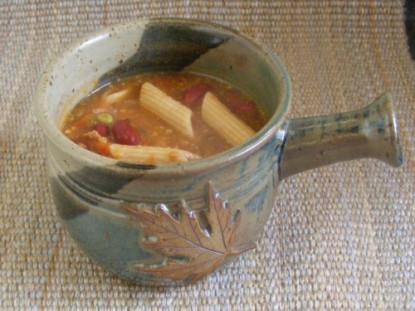This close-up photograph captures a small metal cup, likely stainless steel, designed with a distinct round handle protruding from the right side. The cup is silver, adorned with a light brown, welded leaf detail on its front, and features a small, round pattern encircling it like a stripe. Inside the cup sits a vibrant reddish soup, populated with floating penne noodles, kidney beans, pinto beans, a pea, and various other vegetable ingredients. The cup is placed on a finely woven placemat in light brown with interwoven blue stripes, filling the frame and giving way to a dark background in the upper right corner.